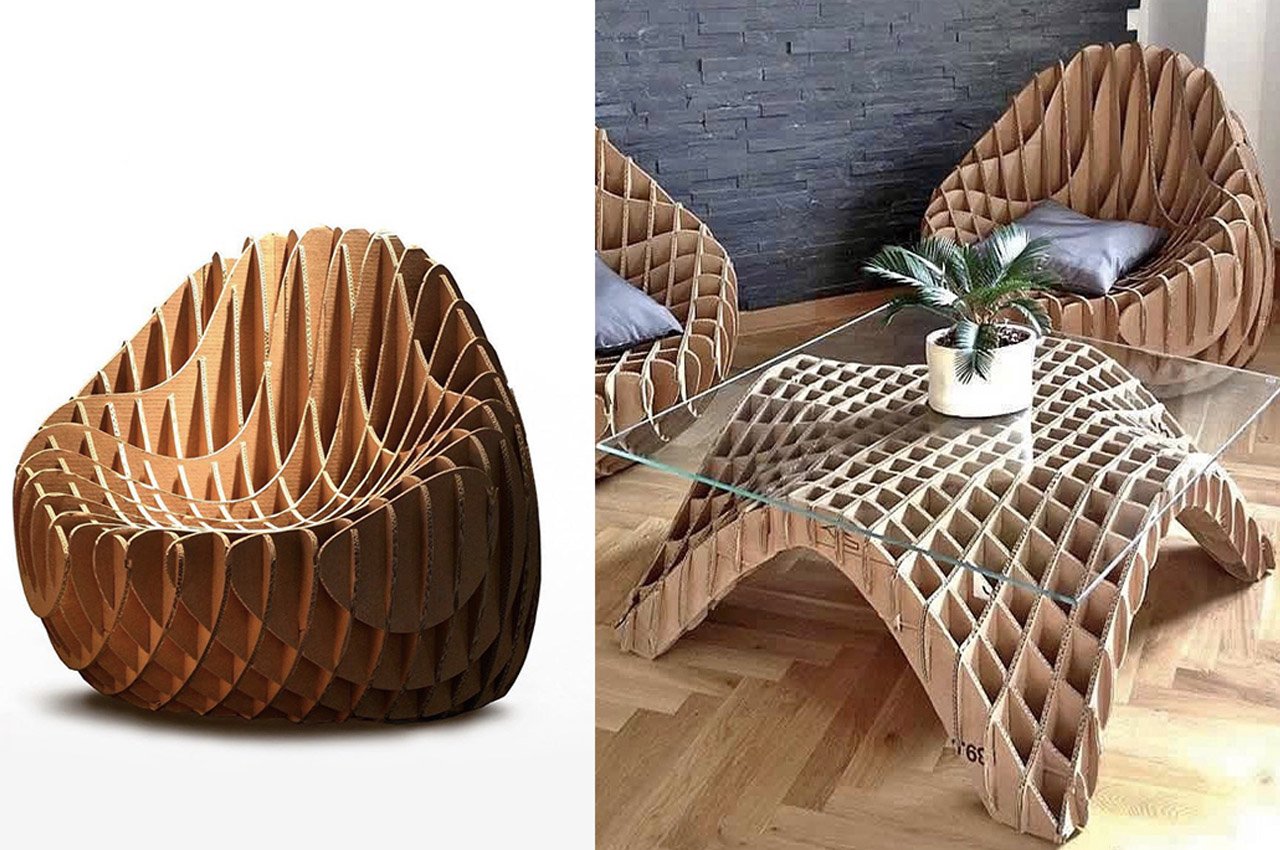The image showcases two photographs positioned side by side, each depicting a modern piece of furniture. The left photograph features a unique chair crafted from light brown cardboard, designed in a honeycomb structure with a hollow interior. The chair's spherical shape is cut off at the top to form a seat, set against a solid white background. The right photograph places the same chair in a real setting: it’s adorned with a gray cushion and accompanied by a matching coffee table composed of interlocking cardboard pieces supporting a square glass top. The background consists of dark gray stone walls and a tan laminate hardwood floor, completing the contemporary aesthetic.